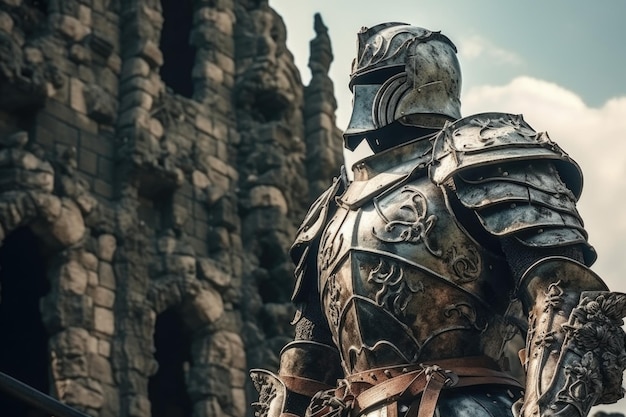The image depicts a towering knight in shining, albeit slightly grimy armor, standing outdoors, likely from a CG-styled video game render. The knight is positioned on the right-hand side of the image, clad in intricately designed, multi-layered shoulder armor, and armored gloves adorned with ornate, floral moldings. The silver chest piece, also with detailed floral patterns, is secured with a brown leather belt fastened around the waist. Additional leather straps are visible on the knight's arms, potentially for securing weapons. The helmet, featuring a long rectangular slit and a pointy mouthpiece, has curved side lines and a thin mohawk-like ridge on top.

In the background on the left side, a tall stone castle made of gray bricks stands against the bright sky, with white clouds visible in the top right corner. The environment is well-lit, providing clear visibility of both the knight and the castle, enhancing the image's overall clarity.